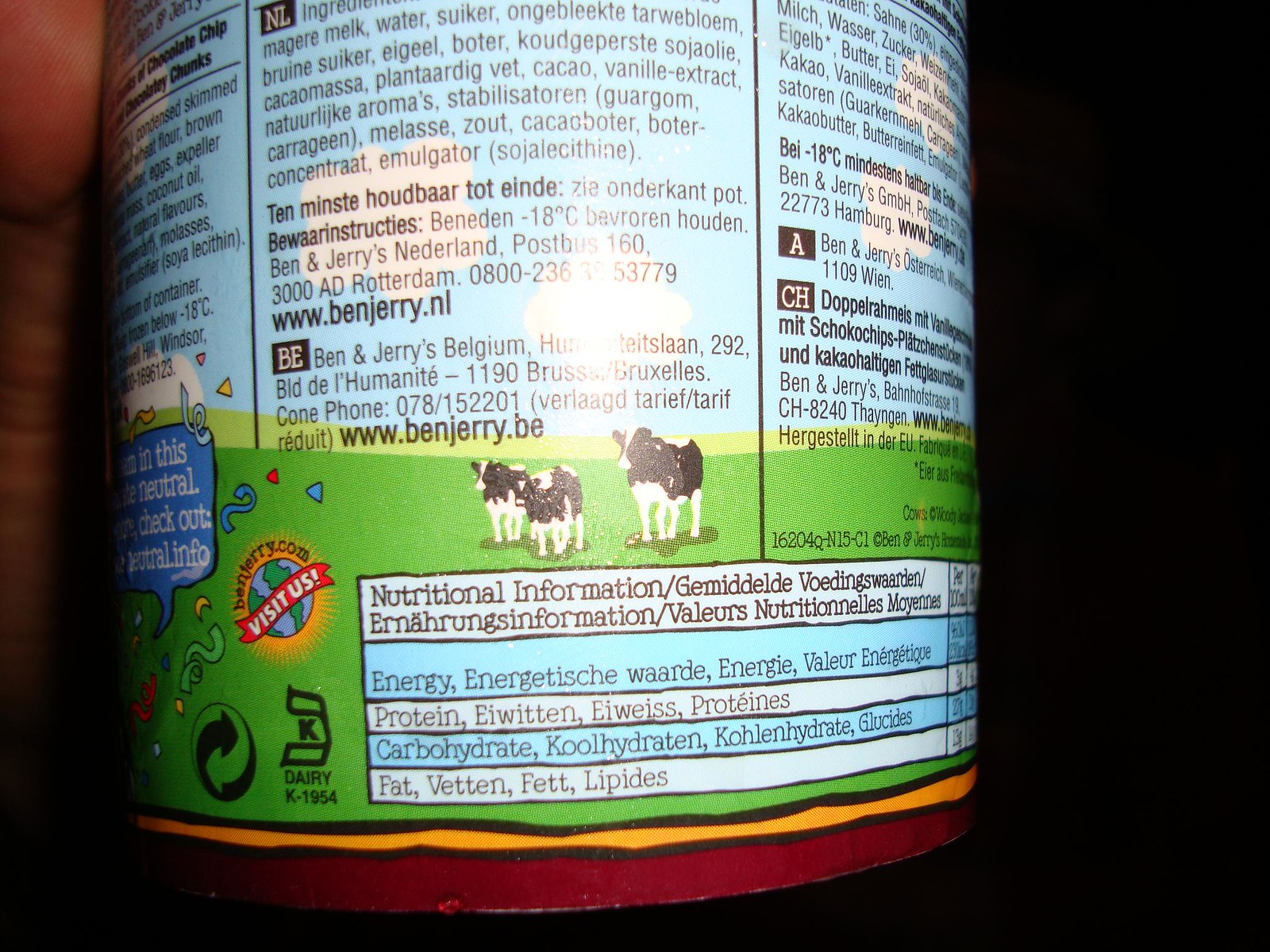The image captures a close-up of the lower section of a Ben & Jerry's ice cream pint label, showcasing a detailed, multi-language nutritional information panel. At the very bottom, a red line is visible, succeeded by a yellow section, and then a green background that features three dairy cows, two small and one large, standing in a grassy field. The nutritional information is presented in multiple languages, listing contents such as Energy, Protein, Carbohydrate, and Fat. Adjacent to this panel, the label includes ingredients, also in multiple languages, along with several icons: a recyclable symbol, a kosher dairy symbol, and a stylized earth with a red ribbon banner saying "Visit Us" followed by "BenJerry.com." The top part of the English section is cut off, and along the left side, there are details mentioning chocolate chip and chocolatey chunks. The label's overall design is indicative of an international version, possibly from Europe.